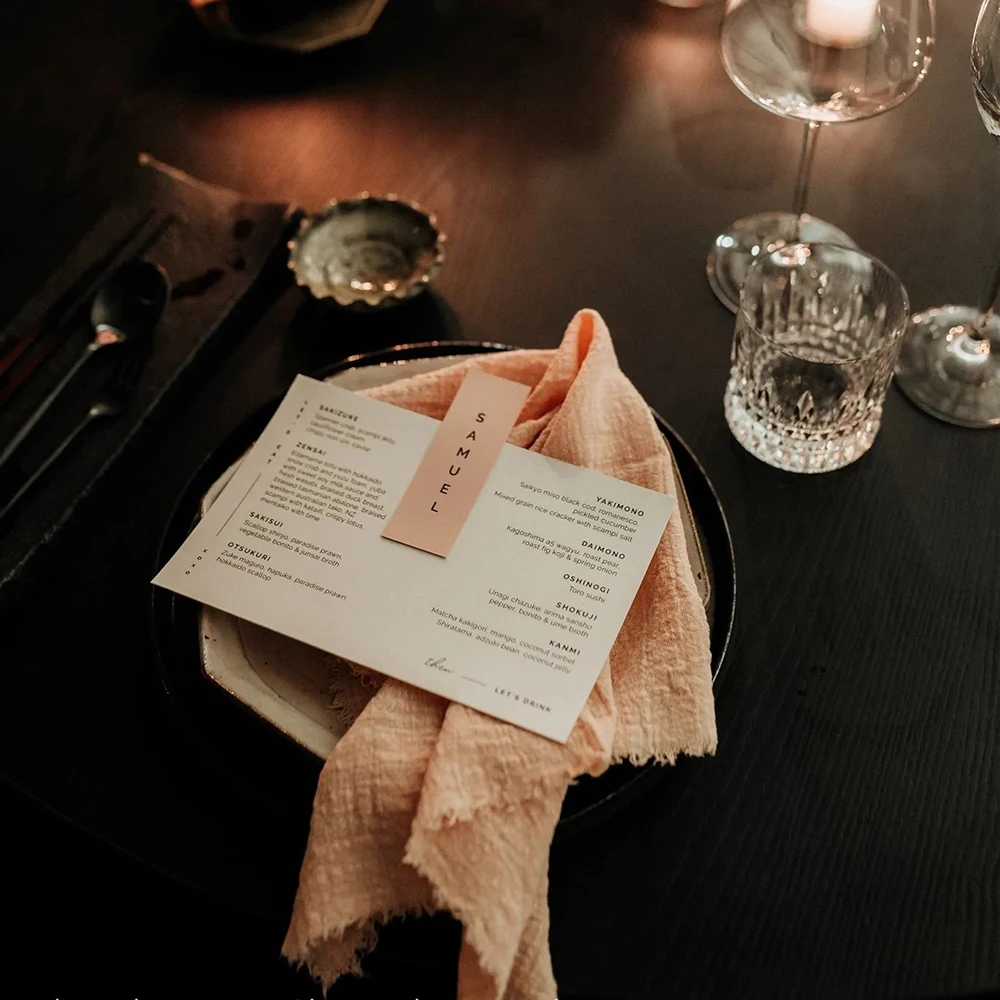In this beautifully arranged overhead shot of an elegant dining setup, a black, sophisticated table serves as the backdrop. At the center sits a black plate holding a delicate peach-colored napkin. On top of the napkin lies a small postcard-like menu with additional details written on a smaller white strip of paper, with the name "Samuel" prominently displayed, possibly indicating a reservation. To the left, just above the plate, there is another small black plate cradling a pair of black chopsticks, a spoon, and a small fork, along with a soy sauce holder next to it. The upper right quadrant features an assortment of crystal glasses, including two intricately designed wine glasses and a short glass, completing this high-class dining table arrangement.